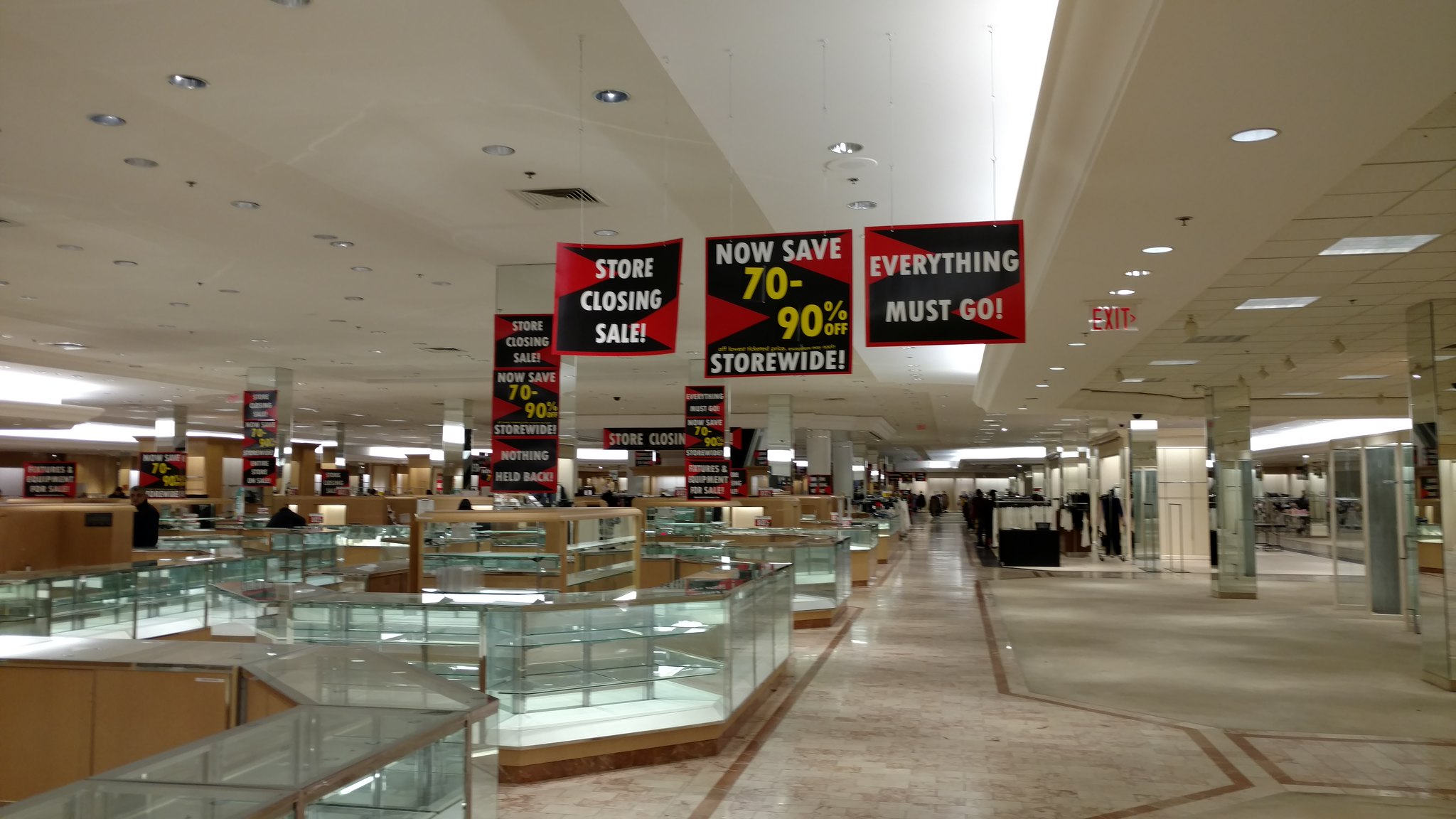This detailed photograph captures the interior of a large department store during a closing sale. Dominating the scene is a long walkway with light-colored tile flooring accented with gold detailing. To the left, numerous empty glass display cases, typically used for jewelry, watches, or fragrances, are illuminated but devoid of any merchandise. On the right, there is a bare section of the floor, possibly cream-colored carpet or white tiles, leading to three steel pillars that suggest the entrance and exit points of the store. Hanging from the white ceiling, which is fitted with fluorescent lights and fire sprinklers running its length, are multiple large banners in red, white, and black colors. These banners announce the store's imminent closure with messages such as "STORE CLOSING SALE," "SAVE 70-90% STOREWIDE," and "EVERYTHING MUST GO." In the background, a few people can be seen milling about, while a sign for an emergency exit is visible on the right side of the image.